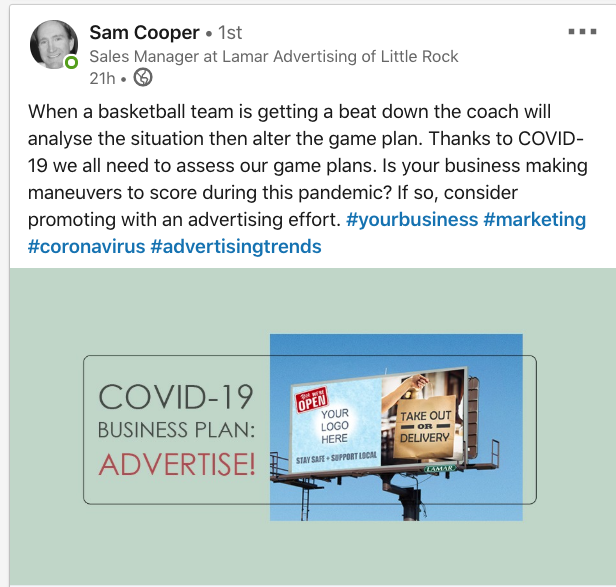In this image, the upper section features a text header by Sam Cooper. On the upper right, there is a three-dot horizontal menu icon, and to the left, a user profile picture signifying the person is online with a green status indicator. The user, identified as a Sales Manager at Lama Advertising of Little Rock, posted this 21 hours ago. The post contains the following text: "Then there are hashtags". The hashtags "#advertisingtrends" are highlighted in blue. 

The background of the top half of the page where the post text is located is white, while the bottom half transitions to a green color. At the bottom of the image, there is a text that reads "COVID-19 business plan advertised," with "advertised" prominently displayed in red and the rest of the text in black. 

On the right side of the image, there is a prominent billboard with the words "Monset High" displayed. The background scenery showcases a blue sky.